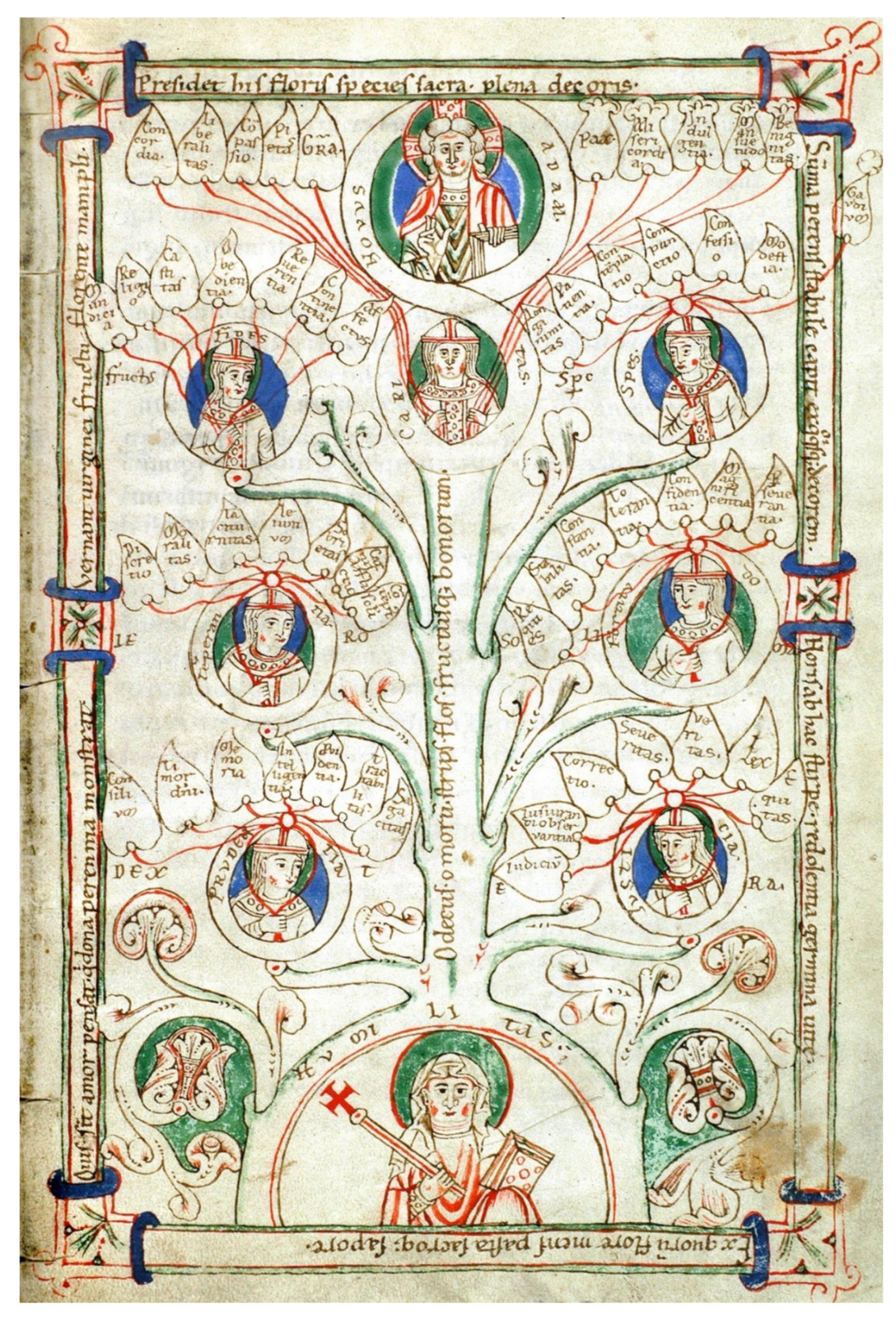This vertical rectangular artwork resembles an ancient piece of parchment paper and features intricate detailing that suggests a religious theme. The image is surrounded by a uniquely divided black border with enigmatic writing that is not in English, arranged so that the text at the bottom is upside down. At the center of the composition is a hierarchical family tree or religious diagram. 

At the top of this tree-like structure is a significant religious figure, possibly Jesus or another revered icon, holding a cross with a gesture resembling a peace sign. The figure is encased in both a blue and a black circle. Branching down from this central figure is a green trunk extending to other animated religious characters, each also encircled in blue and black. Smaller images connect along this tree, symbolizing a lineage or spiritual connection.

The character at the base of the tree, adorned in a red and white robe with a green halo, holds a stick topped with a red iron cross. The entire artwork is peppered with approximately ten distinct religious figures, making it a densely packed, visually rich piece reminiscent of both an old-fashioned poster and a detailed diagram.